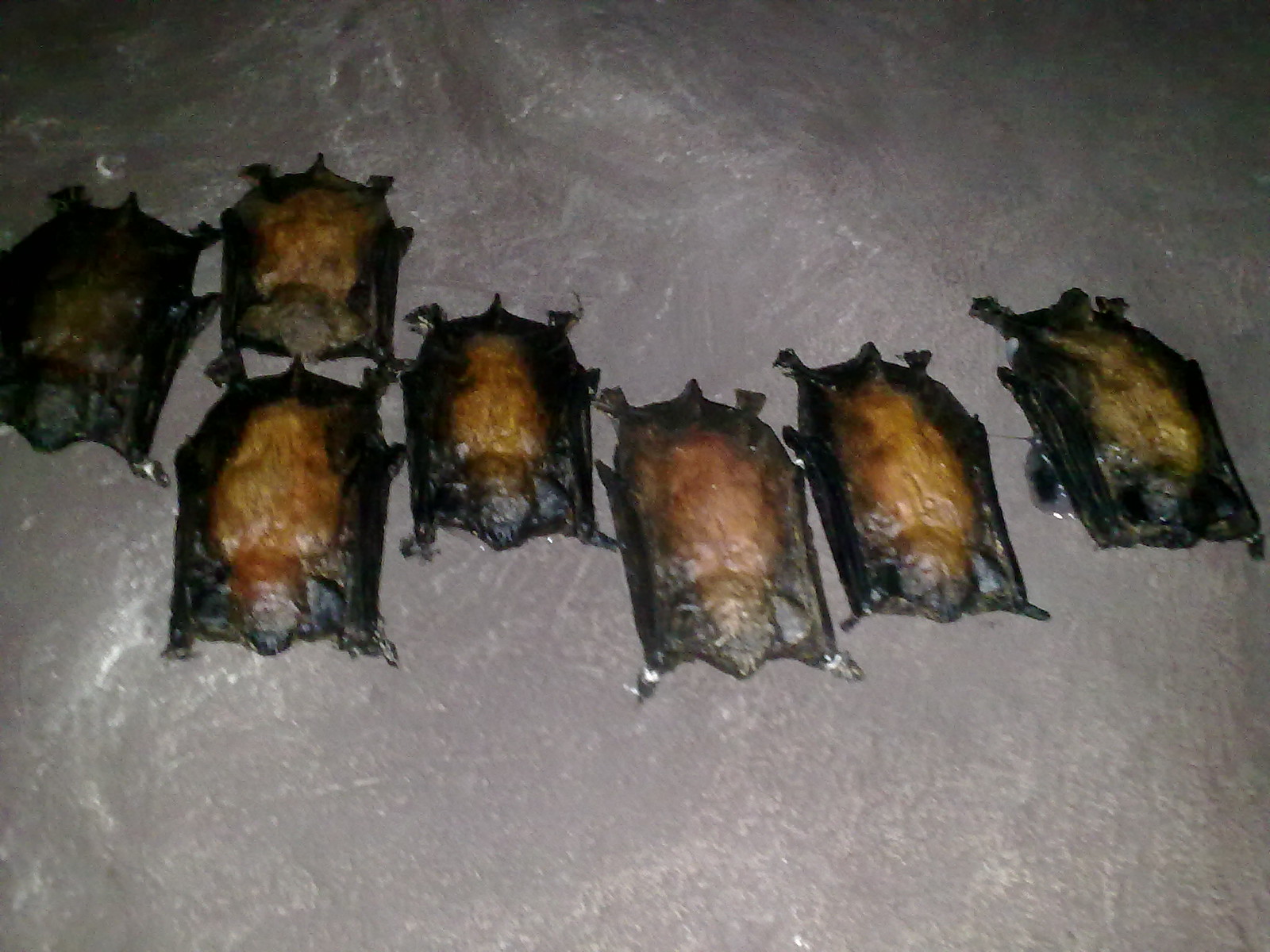This color photograph captures seven mysterious, rectangular-shaped objects lying belly-up on a gray, rock-like surface, possibly bubble wrap or saran wrap. Arranged in a horizontal line, moving from the left side of the photo to the right, these objects feature black edges with golden or tannish centers. Each object appears to have appendage-like extensions, resembling legs, with three at the top and two at the bottom, and what might be a tail and a faint head-like shape. While their exact nature is unclear, they evoke the appearance of small creatures, perhaps bats, creating an intriguing and enigmatic scene.